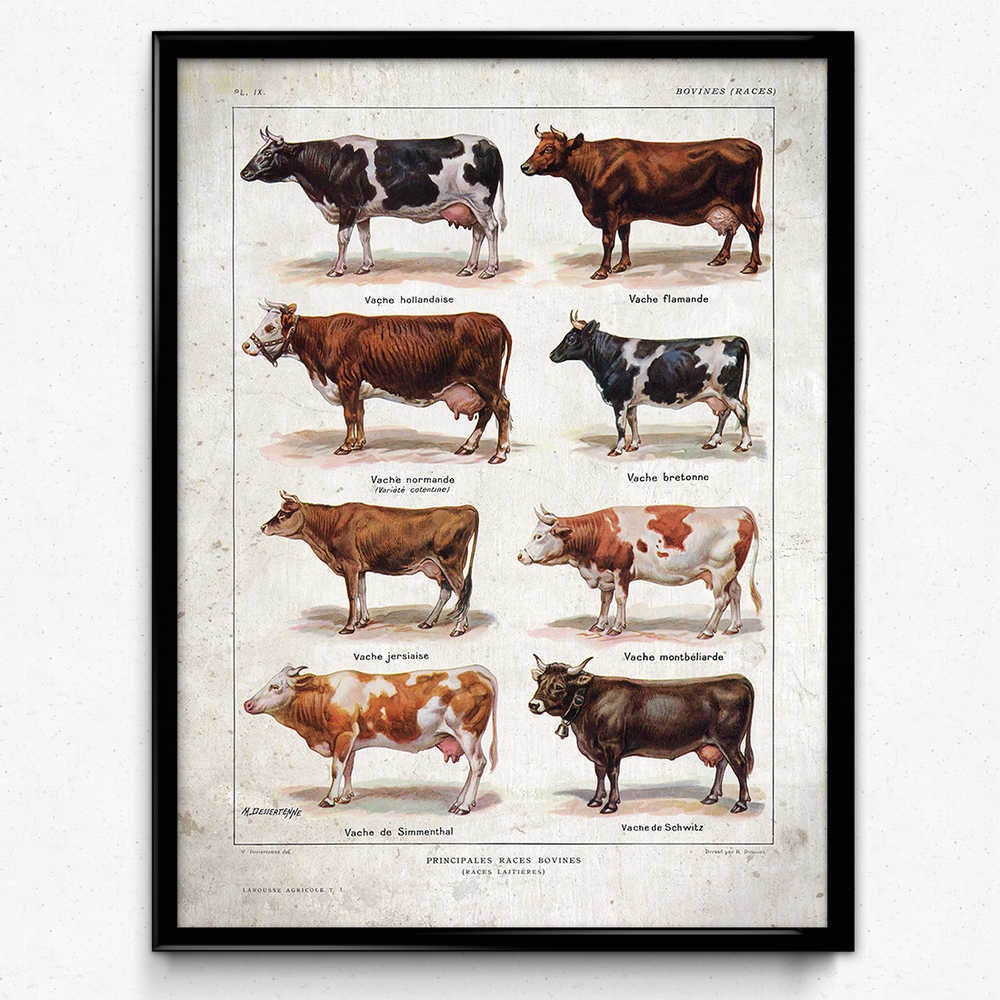The poster titled "Principales Races Bovines" is displayed within a simple black wooden frame, approximately an inch wide. The poster features eight different breeds of cows, organized into two rows of four in a portrait orientation. The background is a dark cream tone, complementing the creamy, spotted black backdrop of the chart.

From left to right, top to bottom, the breeds are as follows:

1. A classic black and white cow positioned in the top left corner.
2. A deep brown cow with horns on the top right.
3. A smaller brown cow with a white face and white underbelly, located below the first cow on the left.
4. A predominantly black and white cow next to it on the right.
5. A light brown cow, thinner and smaller in stature, located beneath the third cow.
6. A larger, white and brown cow, found beside the light brown cow.
7. A muscular, dark brown cow that appears almost leathery, situated in the bottom left, with a distinctive bell around its neck.
8. Adjacent to it is a cow that is mostly white, with notable brown patches on its shoulders, back, and rear end.

The text "Principales Races Bovines" is prominently displayed at the bottom. Additional text is present in the bottom left corner, reading "L'AWOC AGRICOLE" among other words, while the top sections of the poster contain labels such as "PLIX" on the left and "Bovines (Races)" on the right.